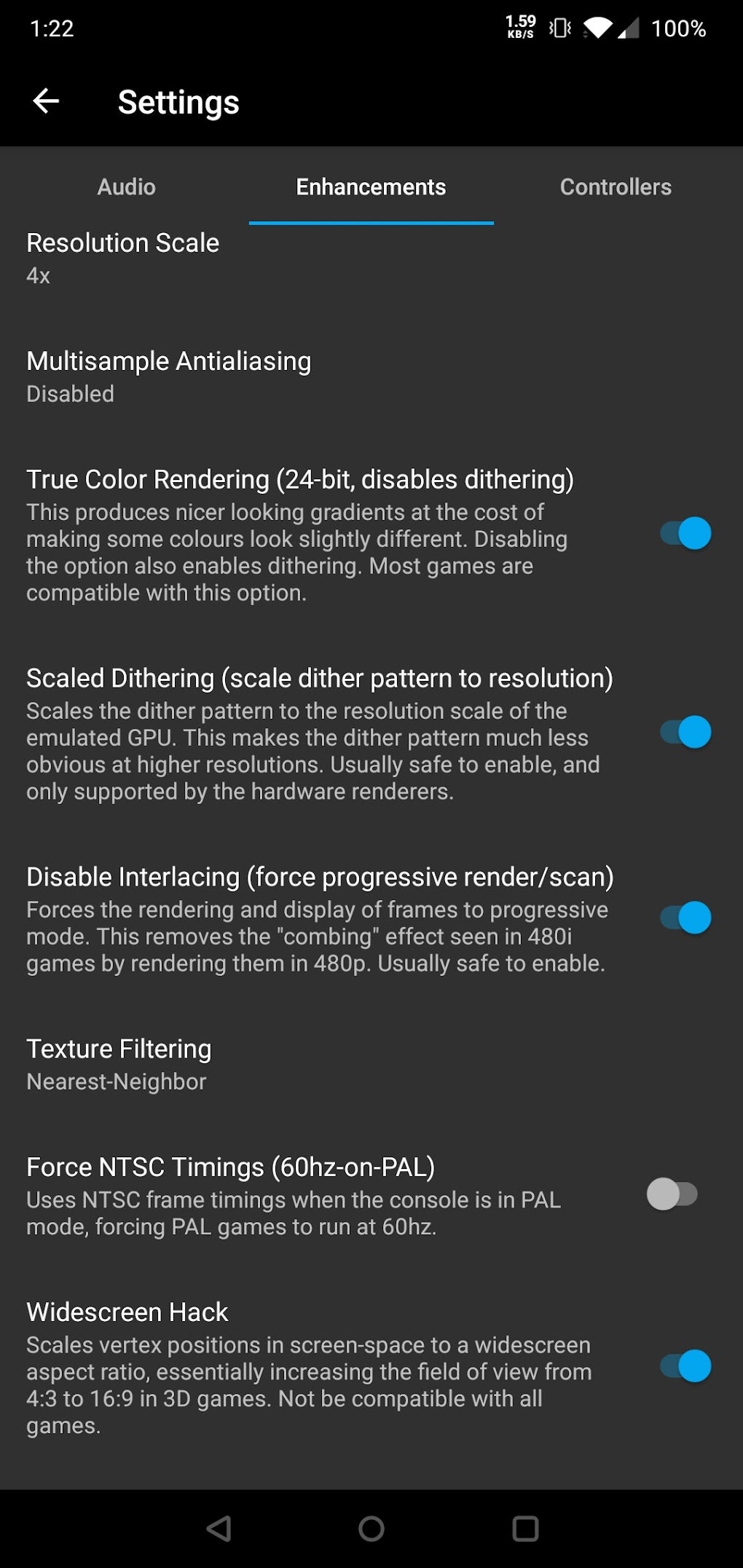Screenshot of a mobile phone screen displaying various settings with a dark-themed interface. At the top, the status bar shows the time (1:22) on the left and the current data transfer rate (1.59 kilobytes per second) on the right. Indicators for the phone's vibrate mode, Wi-Fi (with one bar of signal strength), and a fully charged battery (100%) are visible.

Below the status bar, the title "Settings" is displayed on the left with a leftward arrow icon adjacent to it. Three main headings are listed beneath: "Audio," "Enhancements," and "Controllers." The "Enhancements" tab is highlighted in bright white with an active blue underline, indicating it is currently selected.

Within the "Enhancements" section, the following detailed settings are presented:
1. **Resolution Scale**: 4x
2. **Multi-sample Anti-aliasing**: Disabled
3. **True Color Rendering (24-bit)**: Has a toggle switch on the right, which is enabled and highlighted in blue.
4. **Scale Dithering**: Option to scale the dither pattern to resolution, accompanied by a descriptive note below. This option is also enabled with a blue toggle switch.
5. **Disable Interlacing**: Forces progressive render scan, and this option is enabled with a blue toggle switch.
6. **Texture Filtering**: Set to "Nearest Neighbor."
7. **Force NTSC Timings (60 Hz on PAL)**: This option is grayed out and unselected, with the switch positioned to the left.
8. **Widescreen Hack**: This option is enabled with a blue toggle switch.

The detailed interface displays various sophisticated settings tailored for specific adjustments, enhancing the user experience and offering advanced customization options.